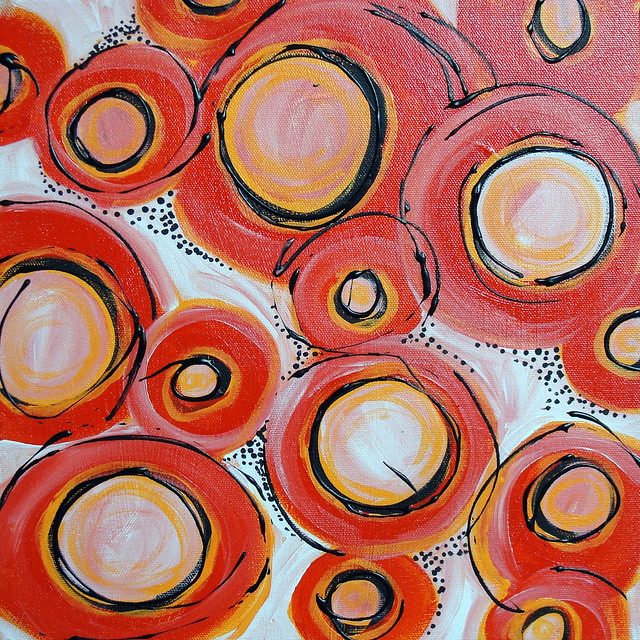The image is a detailed painting in an op art or modern art style, featuring predominantly red, black, pale orange or golden yellow, and white colors. The main design elements are variously sized circles that resemble donuts, drawn in a freehand and abstract manner, resulting in imperfect but visually engaging forms. The largest circles are predominantly red with thin, somewhat sloppily delineated black bands outlining them. Inside each red circle, there is another black circle, which may contain additional colors like pale orange, pink, and white.

These circles overlap and cluster together in random arrangements, creating a dynamic composition. The background is primarily white, speckled with small black dots. In the spaces between the larger circles, the white background provides a contrasting path dotted with these black specks, adding to the overall complexity and texture of the painting. Some circles are very large, while others are medium or small, further varying the visual interest and scale within the piece. The surface texture of the canvas is also subtly visible, reflecting the ambient light, which adds depth to the artwork.